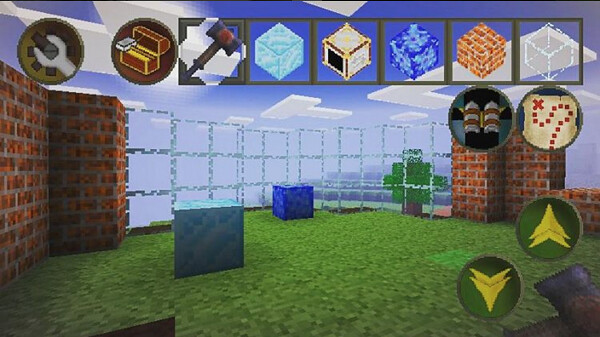The image is a screen capture from a video game, most likely a block-building or construction game similar to Minecraft, likely for a mobile device due to the on-screen UI. The scene is set in a grassy area depicted from a side profile view, framed by tall red brick walls on the left and right. In front of these walls lie two square blocks: a gray block and a blue block positioned slightly behind and to the right. Between the red brick walls in the background are gray, hollow frames that resemble window frames.

The game's interface is filled with various icons. In the foreground, on the lower right corner, are yellow up and down arrows on a green background which suggest interactive commands. The upper portion of the screen is populated with several icons: from left to right, there's a settings (spanner) icon, a treasure chest icon, and a series of six block icons showcasing different materials such as a light crystal blue block, a deeper blue block, a brick-colored block, and a transparent block evocative of glass or frosted outline. These blocks are reflective of the game's building elements seen in the playing area. Additionally, the upper right corner displays map icons, providing navigational assistance within the game. This image illustrates the game's focus on constructing and manipulating walls and blocks within a customizable environment.